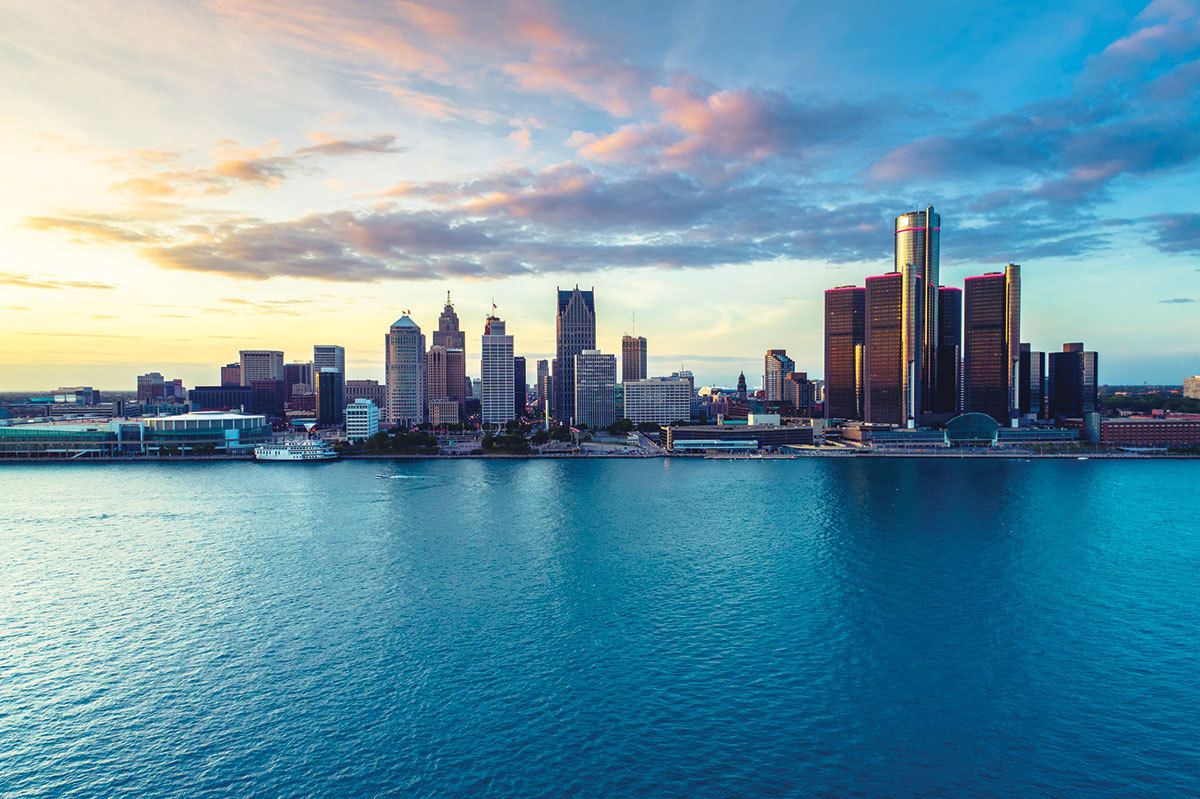The image captures a sprawling cityscape, evocative of Manhattan, situated on an island surrounded by an expansive, still blue body of water. The city's skyline is marked by a gradient of building heights, starting from the left with what appears to be a stadium and lower structures, and progressively advancing to taller skyscrapers adorned with various intricate spires and pointy tops. Towards the far right, there are four similar black buildings surrounding a circular tower. The waterfront includes a small park and a large boat that might be a ferry, with one person skiing in the water. The sky above is a tapestry of soft, pillowy clouds with gentle light shadows, framed by a blue expanse and a hint of yellow sunlight, evoking the time of either a serene sunrise or a peaceful sunset. The city's reflection shimmers on the tranquil water surface, adding to the picturesque quality of the scene.